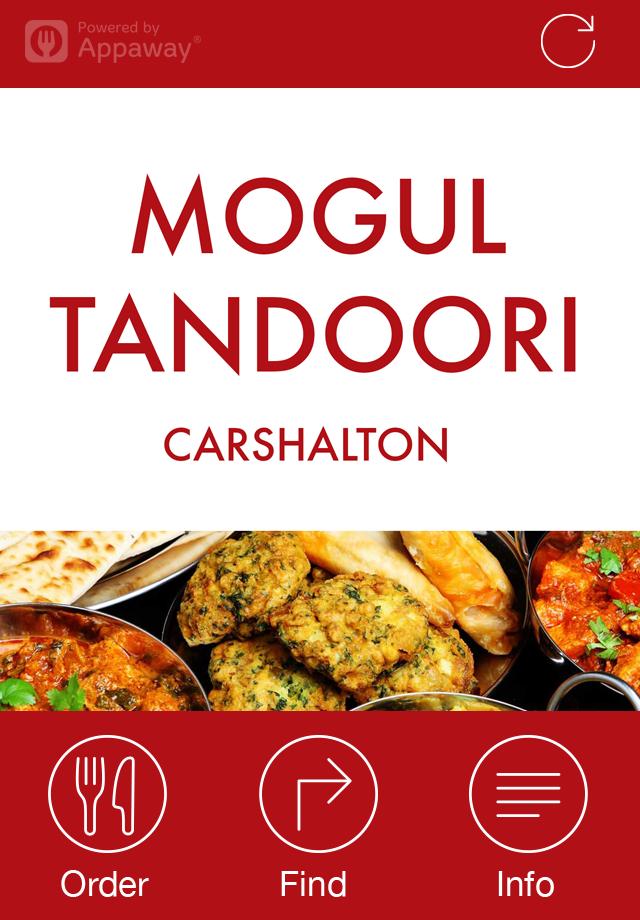The image appears to be the front page of an app or website. At the top, there's a horizontal red border. In the top left corner, there is a faded gray icon resembling a square with the top of a fork inside it. To the right of this icon are the words "powered by Apple Way." On the far right corner, there is a circular refresh symbol—a white circle with an arrow on one end.

The page has a white background. In the center, "Mogul Tandoori" is prominently displayed in red capital letters, with "Carl Shelton" written below it in smaller red capital letters. 

Further down, there is an image showcasing a selection of dishes. The central dish seems to consist of light brown breaded balls with green vegetables inside. To the right, there appears to be a breaded dumpling, and to the left, part of a plate of naan bread is visible. Below the naan, there's a circular silver bowl containing a red, spicy-looking curry with vegetables and meat, garnished with chopped green parsley. On the far right, another bowl of red curry is visible.

Below the image, there's a large red rectangle with three icons inside. On the left, the first icon is a white outline of a circle containing a fork and knife, with the word "order" beneath it. The second icon, in the center, is another white circle outline with an arrow that goes up and then points to the right, labeled "find." The final icon on the right is a white circle with five horizontal lines inside, labeled "info."